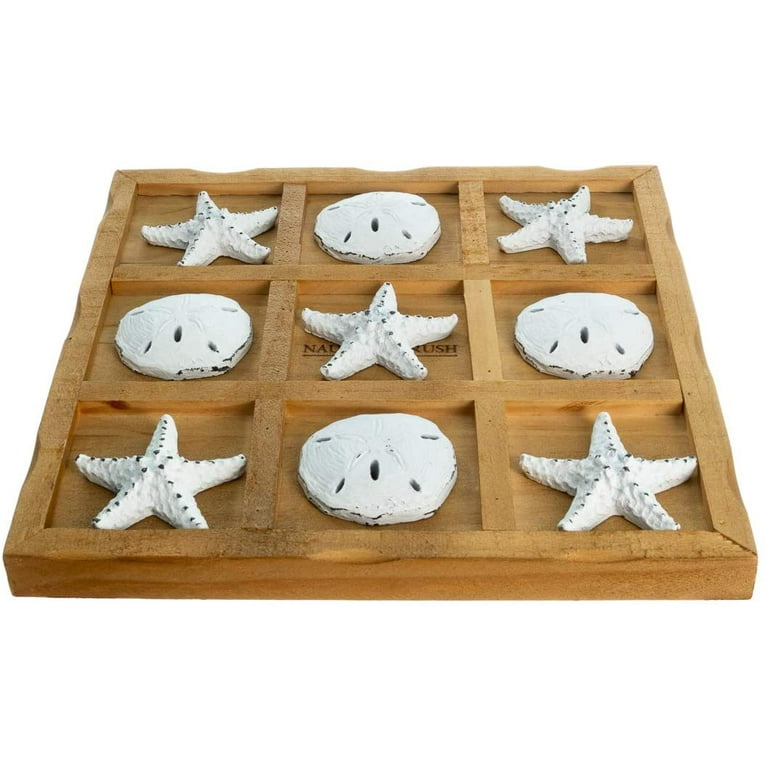The photograph features a decorative, nautical-themed wooden tray, meticulously crafted from light oak wood. This flat, tan square tray is divided into a 3x3 grid, creating nine equal, recessed compartments. Within these compartments, there are white plaster starfish and sand dollars, intended to evoke a beachside motif. The starfish and sand dollars are painted uniformly in pure white, enhancing their contrast against the tan wooden dividers. 

The arrangement of the pieces includes starfish positioned in the upper left, upper right, center, lower left, and lower right compartments. Meanwhile, the sand dollars occupy the upper middle, middle left, middle right, and center squares. Notably, there is one more starfish than sand dollar, with five starfish and four sand dollars in total. The tray is positioned on a flat white background, emphasizing its isolated presentation, which suggests it is likely showcased for decorative or marketing purposes rather than functional gameplay. This detailed arrangement, paired with its oceanic elements, makes it appealing as a decorative piece suitable for a beach house or a nautical-themed setting.